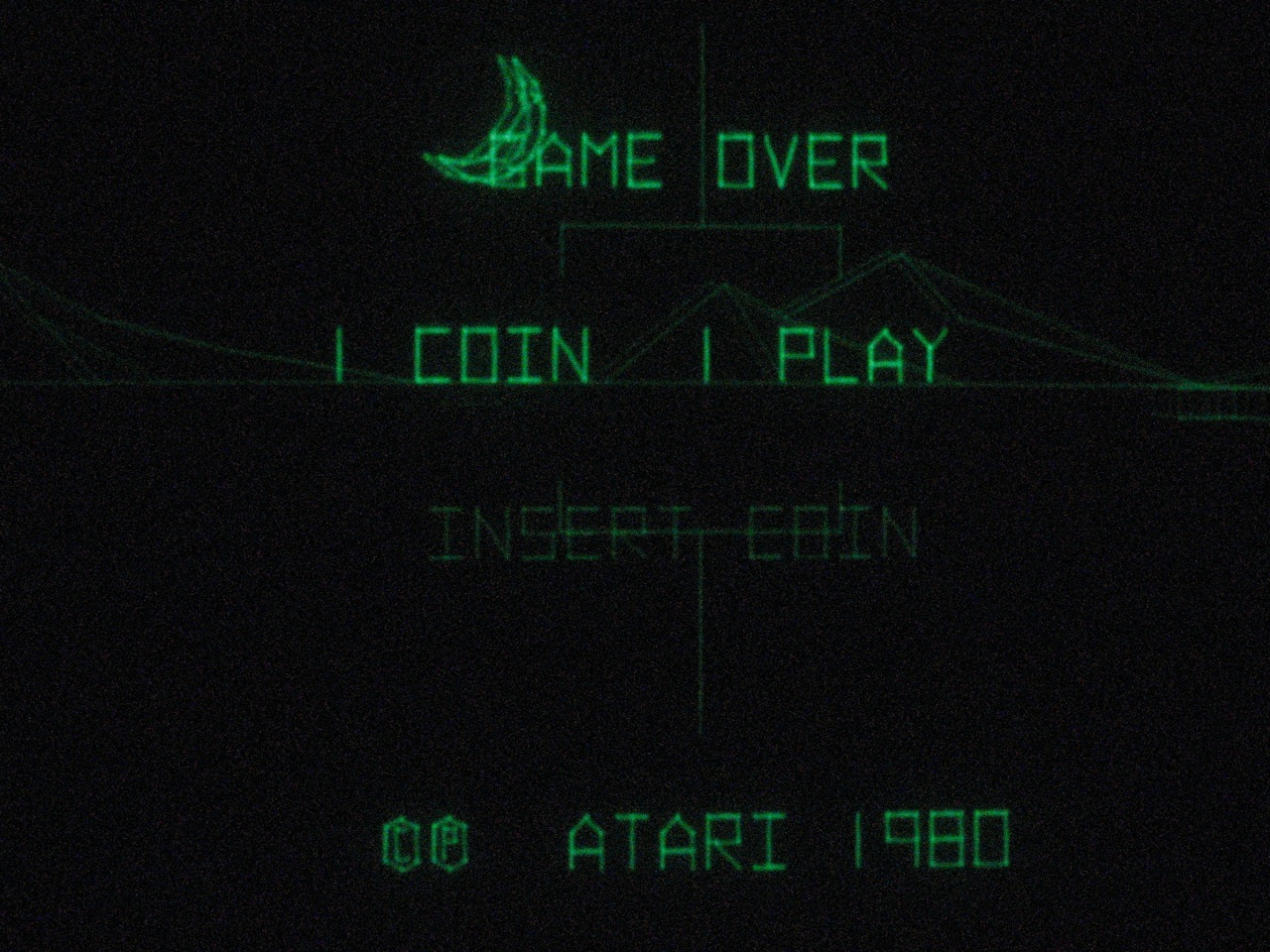This screenshot captures the "Game Over" screen from an Atari game, characterized by its stark black background with neon green text. The phrase "Game Over" is prominently displayed at the top. Below that, the text reads "One Coin, One Play" in a slightly muted green hue, which is almost faded but still legible. Further down, the screen instructs players to "Insert Coin." The bottom of the screen bears a neon green copyright notice: "Atari 1980."

The image quality is somewhat blurry, and there's an intriguing outline that seems to be of mountains behind the "One Coin, One Play" text, adding a subtle depth to the scene. Additionally, a blurry, crescent moon shape hovers near the top, over the "Game Over" text, giving the screen a unique, slightly surreal double-image effect.